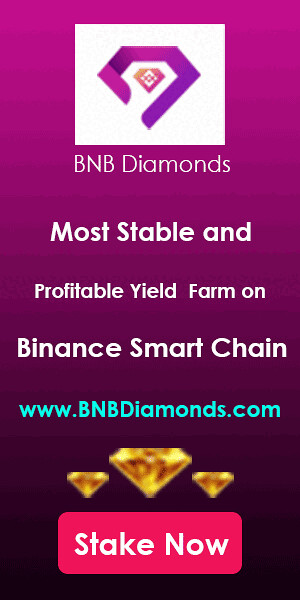The image is a vertically aligned rectangular advertisement with a gradient purple background that transitions from a lighter shade at the top to a very dark purple at the bottom. At the top center, there is a white square featuring a geometric logo resembling an open-sided gem. Below this logo, the text "BNB Diamonds" is written in white. Further down, there are four centered lines of text in white that read "Most Stable and Profitable Yield Farm on Binance Smart Chain". The website address "www.bnbdiamonds.com" appears next in blue letters. Under the URL, the graphic of three gold-colored diamonds is aligned, with the largest diamond in the center and two smaller ones flanking it. At the bottom of the image, there is a small dark pink rectangle containing the text "Stake Now" in white letters. The entire design is a blend of illustration and graphic typography, resembling an internet banner ad.